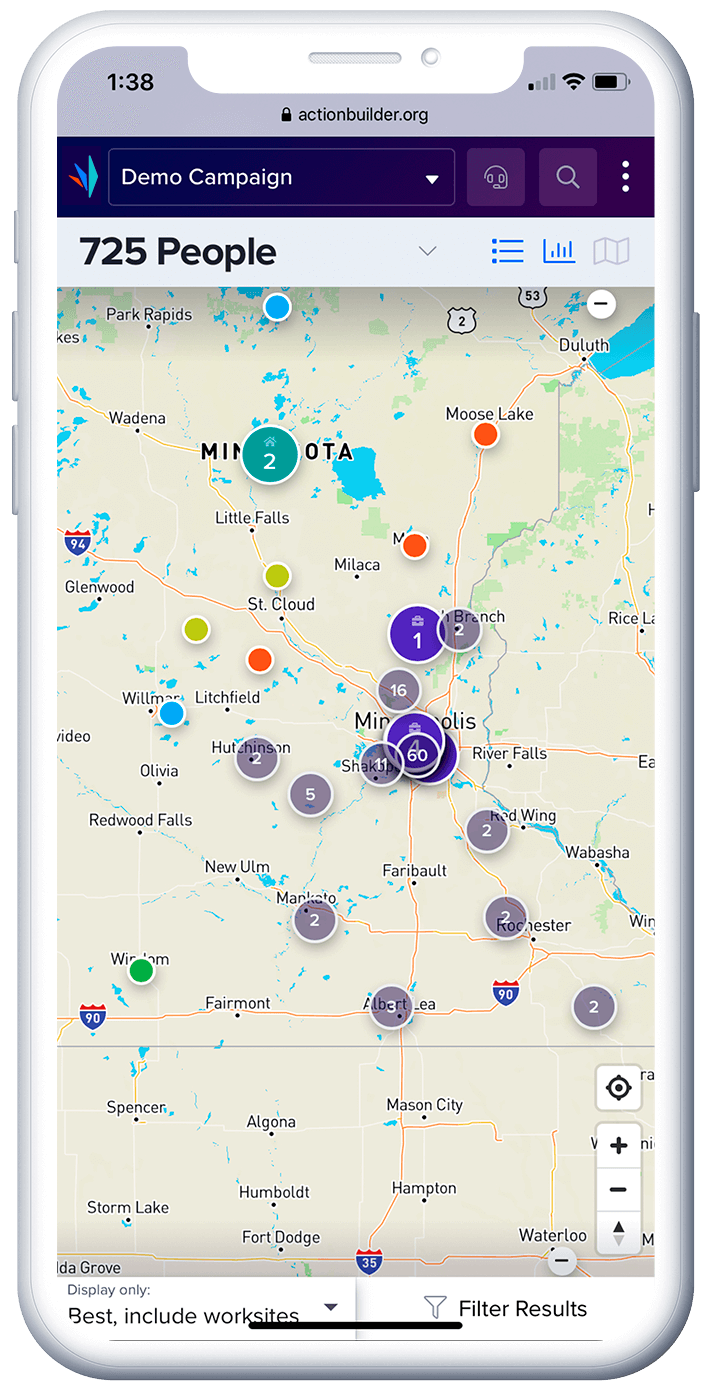The image displays the screen of a smartphone. At the top of the screen, the time reads 1:38, with a weak signal indication but a fully charged battery. Below this, a lock icon appears alongside the URL "actionbuilder.org" on a gray background. 

Central to the image is a vibrant interface featuring a "Demo Campaign" label in a blue box, with colorful strips of paper in teal, blue, and red emerging from behind it. Adjacent to this, there are three icons within a purple box—a pair of earbuds, a magnifying glass, and a vertical arrangement of three dots.

Further down, the screen displays "725 people" next to a map highlighting part of Minnesota. Various buttons and dots are spread across the map; a button marked "60" is prominent, suggesting a higher number of people. The larger buttons seemingly represent more significant numbers of individuals. Most of the dots are gray, with notable exceptions in royal blue, green, and dark blue.

At the bottom, there is a section labeled "Best, Include Worksites," beside a funnel icon that reads "Filter Results." The overall layout combines functional elements and visual markers, indicating a detailed and interactive mapping tool.